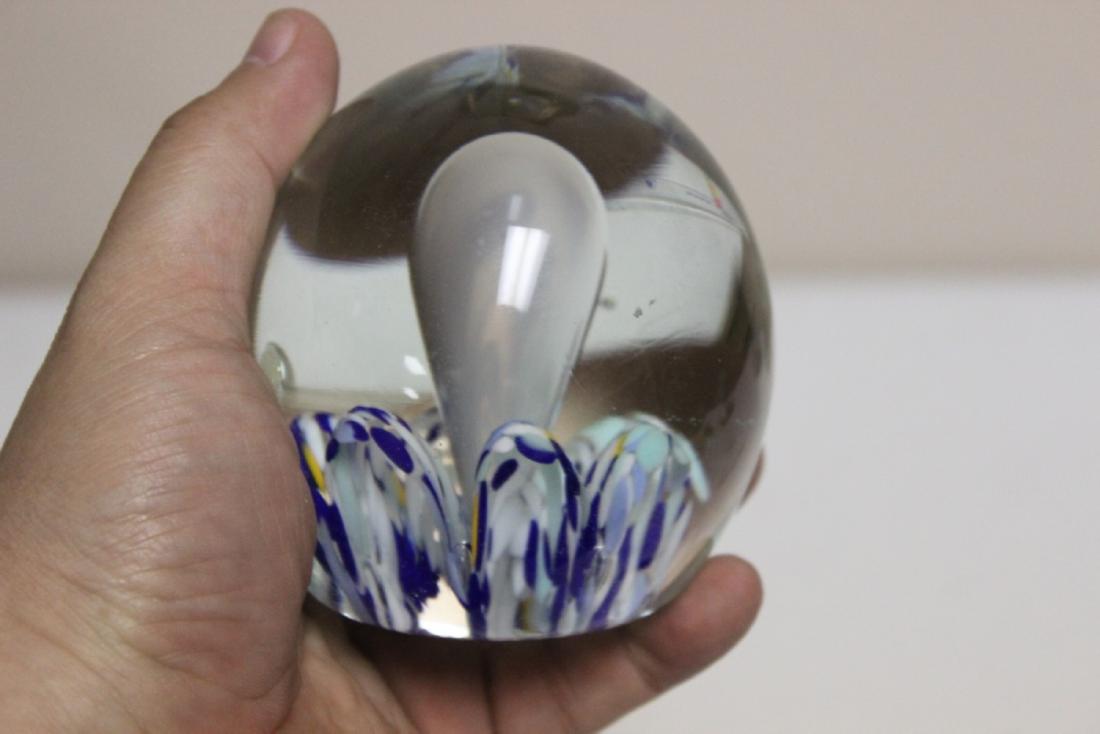The photograph captures a man's hand, emerging from the bottom left of the image and visible from the wrist, clasping a rounded, transparent glass object that could be described as an ornament or a paperweight. His light skin and short nails are evident, along with the plushness of his palm. The glass object, predominantly clear, features an intricate design on its bottom portion—white and deep blue elements forming shapes resembling petals or rope, extending upward in various layers. A central pearl-like structure, reminiscent of an inverted raindrop or a bubble, is prominently placed within the glass. The background is a soft, light hue, combining shades of white and beige, creating a neutral and calming backdrop.